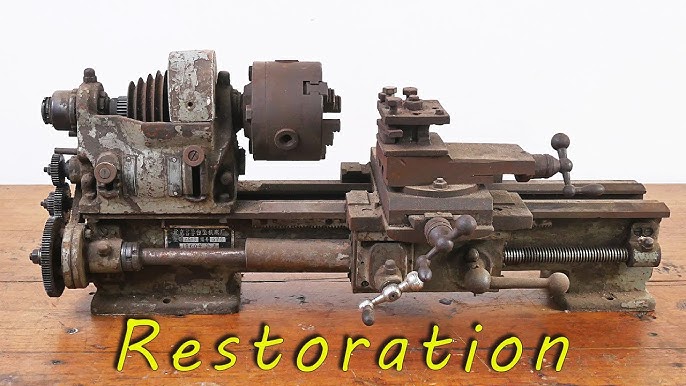This detailed photograph captures a large, antique-looking piece of machinery, likely used for woodworking or wood restoration. The heavy, solid metal tool, characterized by its brownish, rusted appearance, is adorned with various turning knobs, dials, rods, and clamps, reflecting its intricate functionality. Situated on a lengthy brown wooden table, the machinery is set against a stark white background, emphasizing its detailed structure. There's a black and white company tag on the bottom left-hand side, adding to its vintage appeal. Prominently displayed in yellow block lettering on the table is the word "restoration," highlighting the tool's purpose. The machinery seems designed to hold and spin blocks of wood, operated by its numerous gadgets and turning handles.